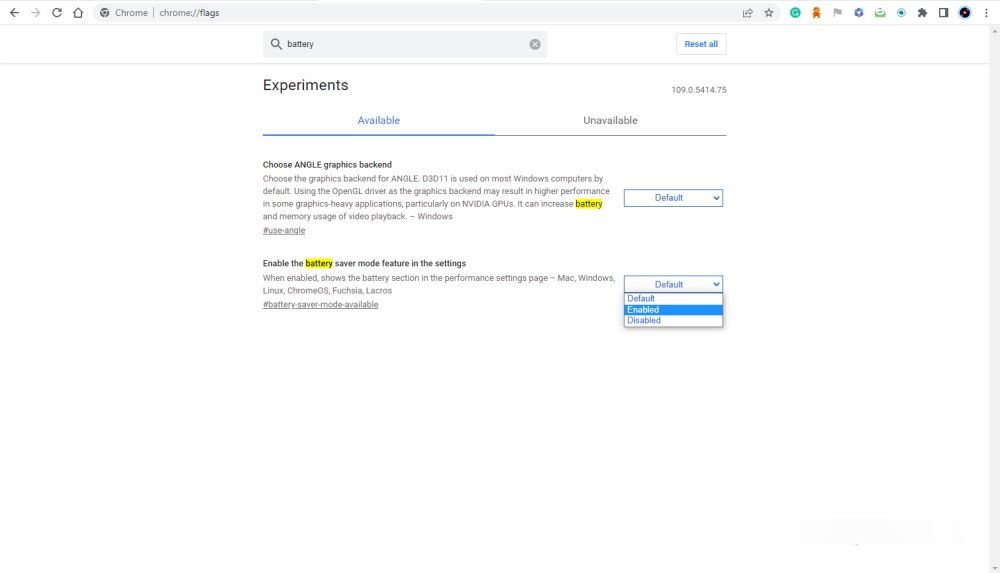**Detailed Caption:**

The screenshot depicts a user navigating the Google Chrome browser on a desktop or laptop. The browser window is open to a page with a white-background header at the top. Central to the header is a search bar with a light gray background, designed in a rectangular shape. On the far left of the search bar, there is a dark gray icon of a magnifying glass, symbolizing the search function. Adjacent to the right of the magnifying glass, in small gray text, the word "battery" is visible. At the far right of the search bar, a gray circular icon with a white 'X' in the center is present.

To the immediate right of this search bar, there is an icon featuring a white background that seamlessly blends with the overall page background. It is enclosed within a light gray rectangular border. Centered within this icon, in bold blue lettering, are the words "Reset all."

Beneath the header, a light gray line acts as a divider, stretching across the page. Below this line, positioned towards the left, the word "Experiments" is written in bold black text.

Two tabs, labeled "Available" and "Unavailable," are situated beneath the "Experiments" section. The "Available" tab is selected and highlighted in blue with a blue underline, denoting its active status. The "Unavailable" tab, appearing towards the right, is in gray with a gray underline. In the top right corner of the "Unavailable" tab, in small gray font, the version number "109.0.5414.75" is displayed.

Below the active "Available" tab, small bold black text reads "Choose ANGLE graphics backend." A descriptive paragraph in small black text is present underneath, with the word "battery" highlighted in yellow for emphasis. To the right of this paragraph, a drop-down menu with a blue border is visible. Inside the drop-down menu, the word "Default" is displayed in blue text, accompanied by a downward-pointing blue arrowhead, indicating it as a selectable menu.